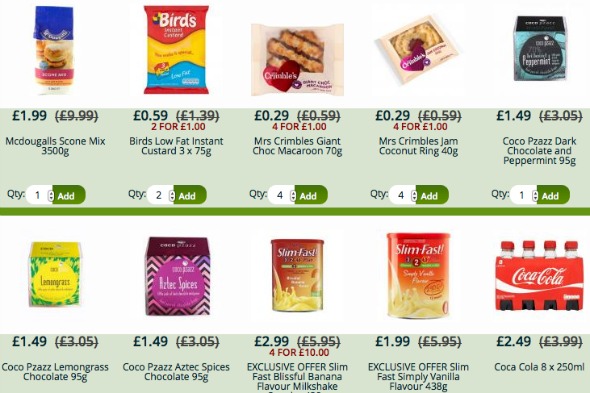This is an image showing a selection of food items available for purchase on a website. Each item listing includes a picture, pricing details, and options for quantity selection.

*Top Row Items:*
1. **McDougal's Scone Mix** - 3,500 grams, priced at £1.99 (regular price £9.99). Quantity option available.
2. **Byrd's Low-Fat Instant Custard** - Pack of three, 75 grams each, priced at £0.59 (original price £1.39), or two packs for £1. Quantity option: Two for £0.29 or four for £1.
3. **Mrs. Crimble's Giant Chocolate Macaroon** - 70 grams, priced at £0.29 or four for £1. Four items added to the cart.
4. **Mrs. Crimble's Jam Coconut Ring** - Price not specified due to incomplete information; it seems to involve a quantity of four items.
5. **Cocoa Paws Dark Chocolate & Peppermint** - 95 grams, priced at £1.49.

*Bottom Row Items:*
1. **Cocoa Paws Lemongrass Chocolate** - 95 grams, priced at £1.49.
2. **Choco Pazza Aztec Spices Chocolate** - Priced at £2.99 or four for £10.
3. **Exclusive Authors Film Fest Blissful Banana Flavor Milkshake** - 1.99 pound, the precise serving size is not specified.
4. **Exclusive Authors Film Fest Simply Vanilla** - 4.38 grams, priced at £1.99.
5. **Coca-Cola** - Pack of 8, 250 milliliters each, priced at £2.49.

This detailed caption encapsulates the variety of products available on the food website, including price points and quantity options for each item.